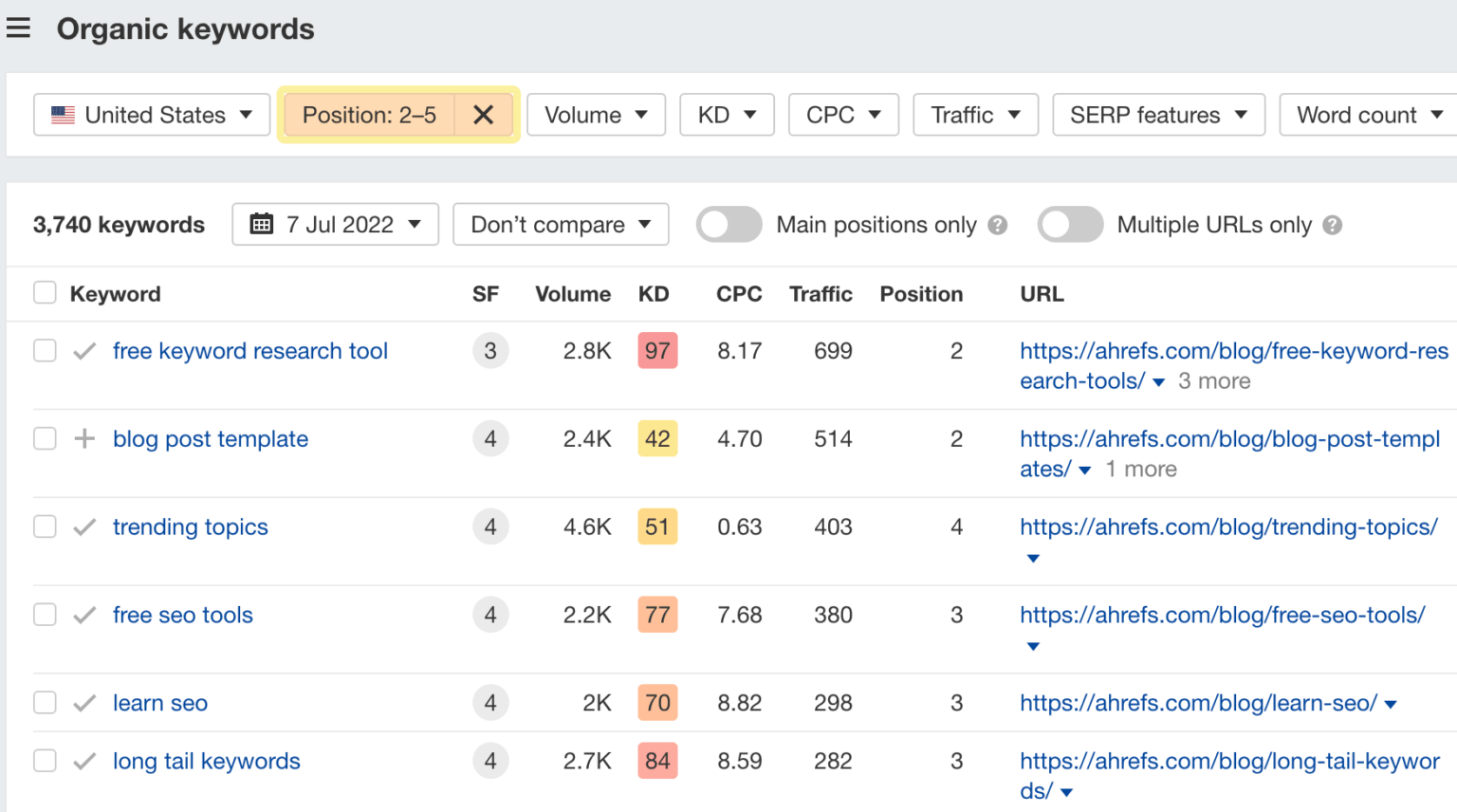A detailed view of a keyword tracking webpage designed for optimizing search engine rankings. The page is titled "Organic Keywords" and features a three-line context menu on the left-hand side for easy navigation. At the top, there are small square labels representing different keywords, each with an associated United States flag, arranged with positions two to five highlighted in yellow to indicate selection.

The columns on the page are labeled as follows:
- **KD**: with a context menu for keyword difficulty.
- **CPC**: with a context menu for cost per click.
- **Traffic**: includes a down arrow for additional sorting options.
- **SERP Features**: with a context menu displaying search engine results page features.
- **Word Count**: with a context menu for filtering by word count.

The page displays detailed metrics:
- **3,740 keywords** tracked as of **July 7, 2022**.
- Options like "Don't compare" (context menu available), "Main positions only" (not selected), and "Multiple URLs only" (not selected).

Under the keyword research section, there are specific details for one keyword:
- **SF**: 3
- **Volume**: 2.8K searches
- **KD**: 97 (in red, indicating high difficulty)
- **CPC**: $8.17
- **Traffic**: 699 visits
- **Position**: Number 2 
- **URL**: "http://A4Fs/blog/free-keyword"

Highlighted keywords include:
- Free Keyword Research Tool
- Blog Post Template
- Trending Topics
- Free SEO Tools
- Learn SEO
- Long Tail Keywords

The numbers accompanying these keywords indicate various metrics, potentially linked to their search volume, keyword difficulty, and other SEO-related data, aimed at maximizing the website's visibility and performance in search engine results.